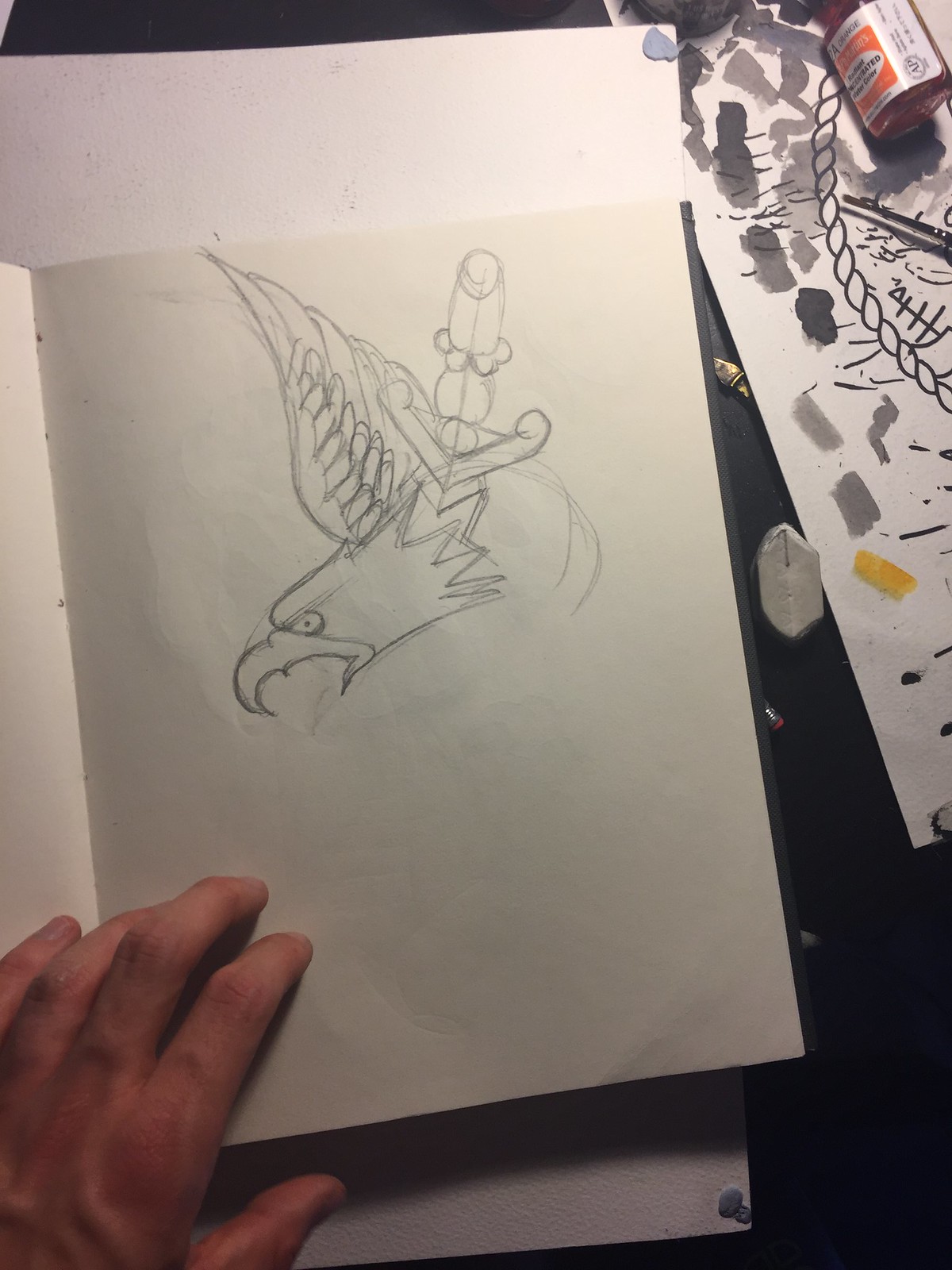In this color photograph, we see a drawing of a bird, resembling a parrot or eagle, on a white sheet of drawing paper, held at the bottom left corner by an adult's hand. The image is taken from a slightly elevated angle, displaying the sketchbook centered and slightly to the left. The bird's head is detailed with a curved beak, beady eyeball, and partial wings, poised as though gripping a pole. Surrounding the sketchbook, we observe additional artistic elements: to the right lies another artwork featuring diverse ink splotches in yellow, gray, and black, alongside a brown bottle with a white and orange label. The scene unfolds atop a black desk, adding contrast to the creative chaos. The layering of papers, the sketchbook fold, and the scattered art supplies, including a tube of paint with a white label and red markings, capture the essence of an artist’s workspace, hinting at a dynamic interplay between adult and child creativity.